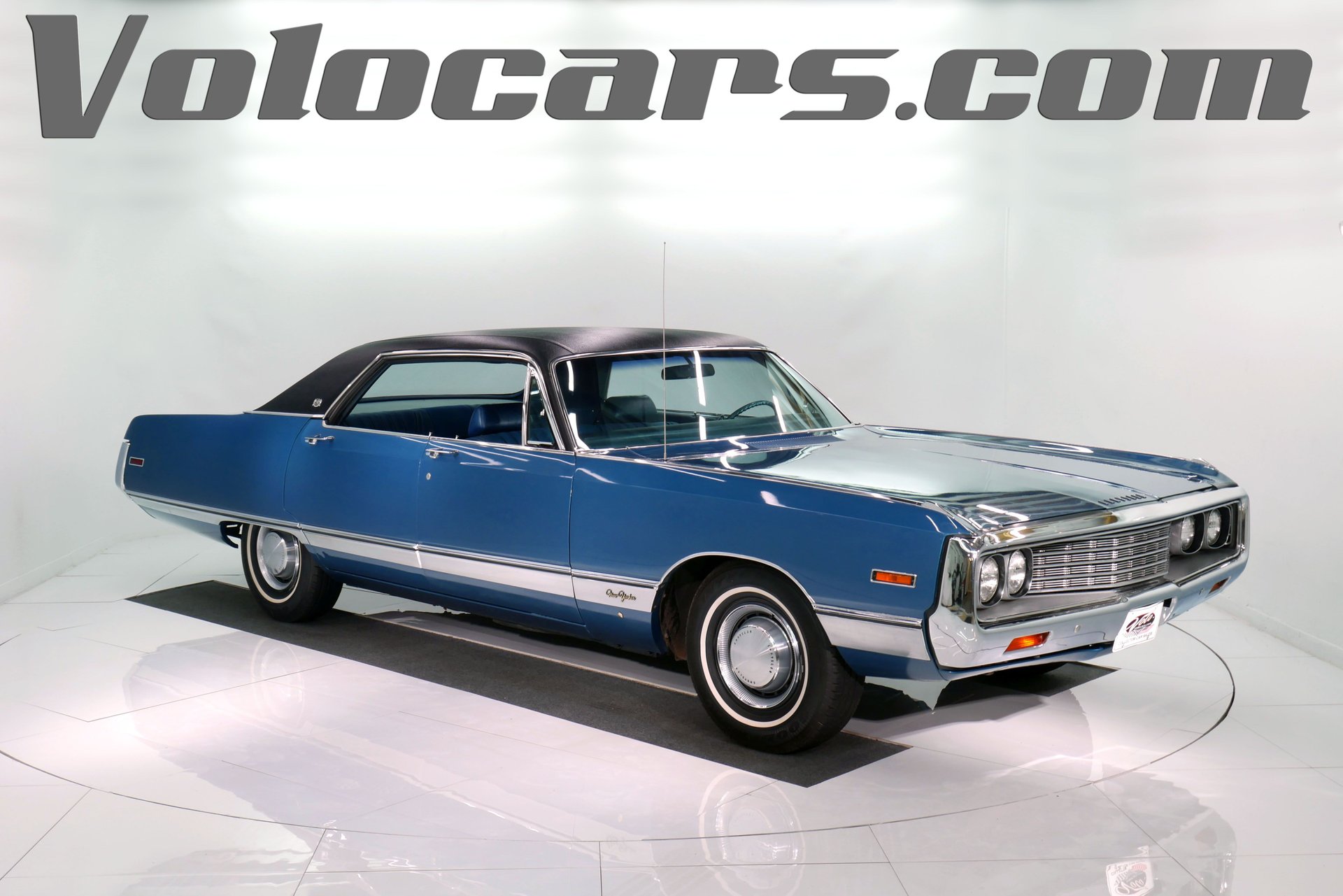The vertical poster features a vintage 1960s convertible prominently displayed against a light gray, reflective background. The car is angled, facing to the right, showcasing its deep blue body accented by a sleek white stripe along the lower section. It has a distinctive black roof and a single large window on each side of its two double doors. The front facade of the car is highlighted by a three-line silver grille centered between two sets of headlights, one pair on each side. The grille and headlights are complemented by black tires with classic white-ringed walls. The reflective floor mirrors the car's details, adding depth to the image. At the top of the poster, in dark gray letters, "volocars.com" is prominently displayed. An old-fashioned radio antenna extends from the right-hand fender, emphasizing the car's vintage appeal. The car appears to be positioned on a turntable for full 360-degree viewing.